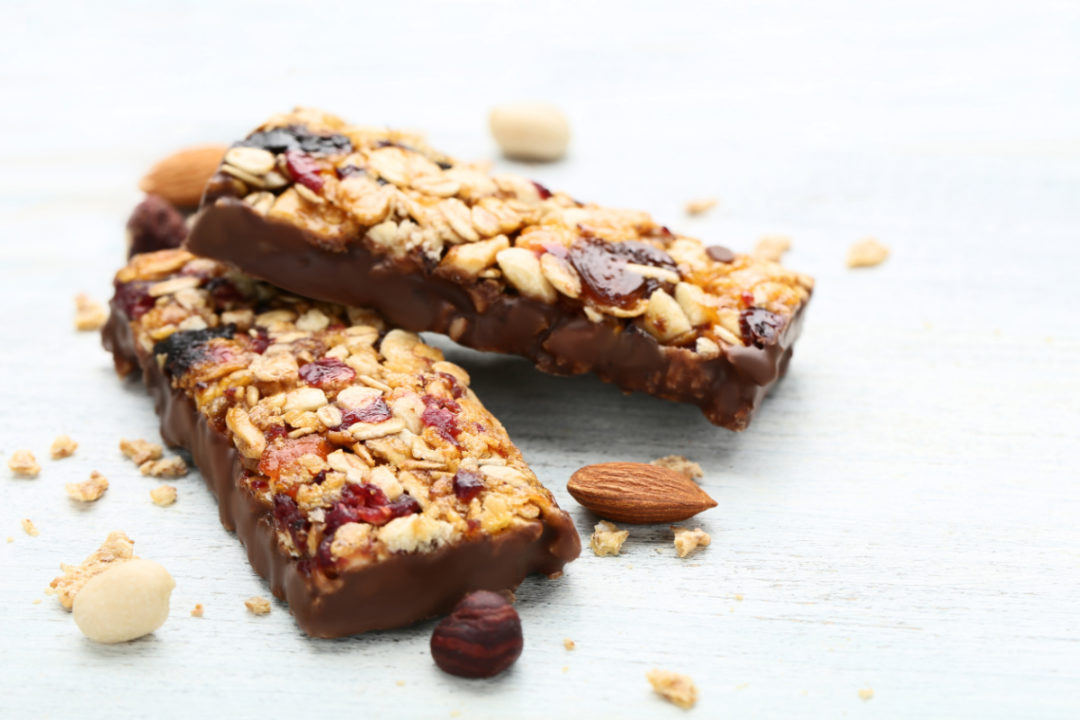The image features a professionally taken, close-up photograph of two granola bars slightly overlapping on a light bluish-gray or whitish wooden surface with black lines running horizontally. The bars are intricately molded together, incorporating a variety of nuts, including whole almonds, peanuts, and smaller seeds like flaxseed. The mix also includes visible cranberries, raisins, oats, and apricots. Both granola bars are partially coated in milk chocolate, with one of them additionally drizzled in chocolate along the lower half. A whole almond is prominently placed at the center of the frame. In addition to the granola bars, the surface also holds scattered loose oats and both white and chocolate-covered raisins. The careful composition and natural lighting highlight the textures and ingredients, providing a vivid and appetizing visual.